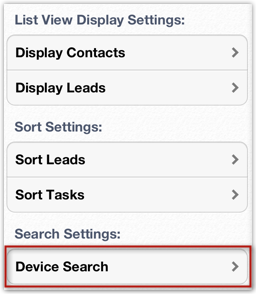The interface screenshot displays settings for a list view in a minimalist design. At the top, the title "List Views Display Settings" is presented in a light gray font. Below the title, two interactive boxes are shown. 

The first box reads "Display Contacts," with both 'D' and 'C' capitalized, in bold black text. Beside this label, there is an arrow indicating an option to expand or interact with the settings further. Directly below, a similar box labeled "Display Leads" also appears in bold black text with the same expandable arrow.

Under these settings, there is another section in gray labeled "Sort Settings:". This section includes options such as "Sort Leads" with a right-arrow for further actions and "Sort Tasks" listed directly beneath.

Further down, a "Search Settings" label in light gray is positioned, followed by a prominently highlighted option. This last option, "Device Search," is encased in a noticeable red box, suggesting it is either the currently selected item or intended for immediate attention.

Overall, the screenshot presents a basic yet functional display settings interface with clearly delineated options for managing contacts, leads, sorting tasks, and search functionalities.